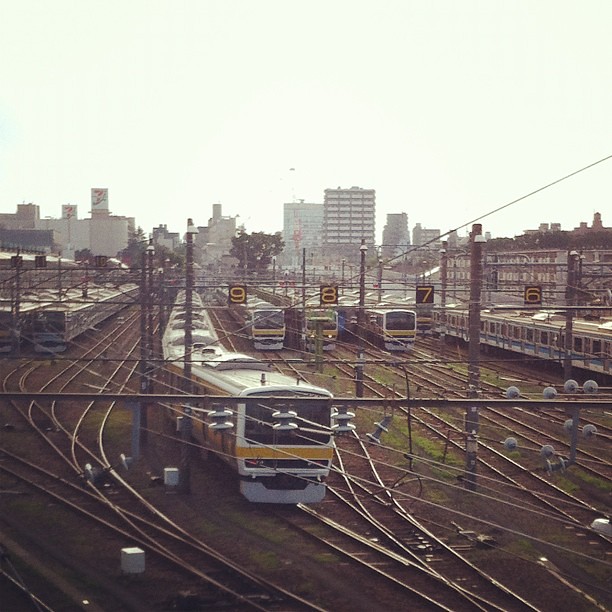This vintage photograph depicts a bustling train station in Japan, characterized by its muted colors and older train models. The station houses up to nine tracks, clearly marked with numbers, and features trains predominantly colored white with yellow sides and fronts, lined up and facing forward. Track numbers six, seven, eight, and nine are visible, with the train on the ninth track in motion. To the right, three to four sturdy dark apartment buildings with white shutters stand against a backdrop of high-rise buildings, indicating a large city skyline. On the left side, an industrial area is noticeable with fewer windows and balconies. The ground between the tracks shows patches of grass amidst the dirt and rails, while streetlights dot the station. Additionally, a unique white train with light and dark blue stripes adds contrast to the scene. The overall atmosphere suggests a late afternoon setting with a hazy sky, enhancing the nostalgic feel of the image.